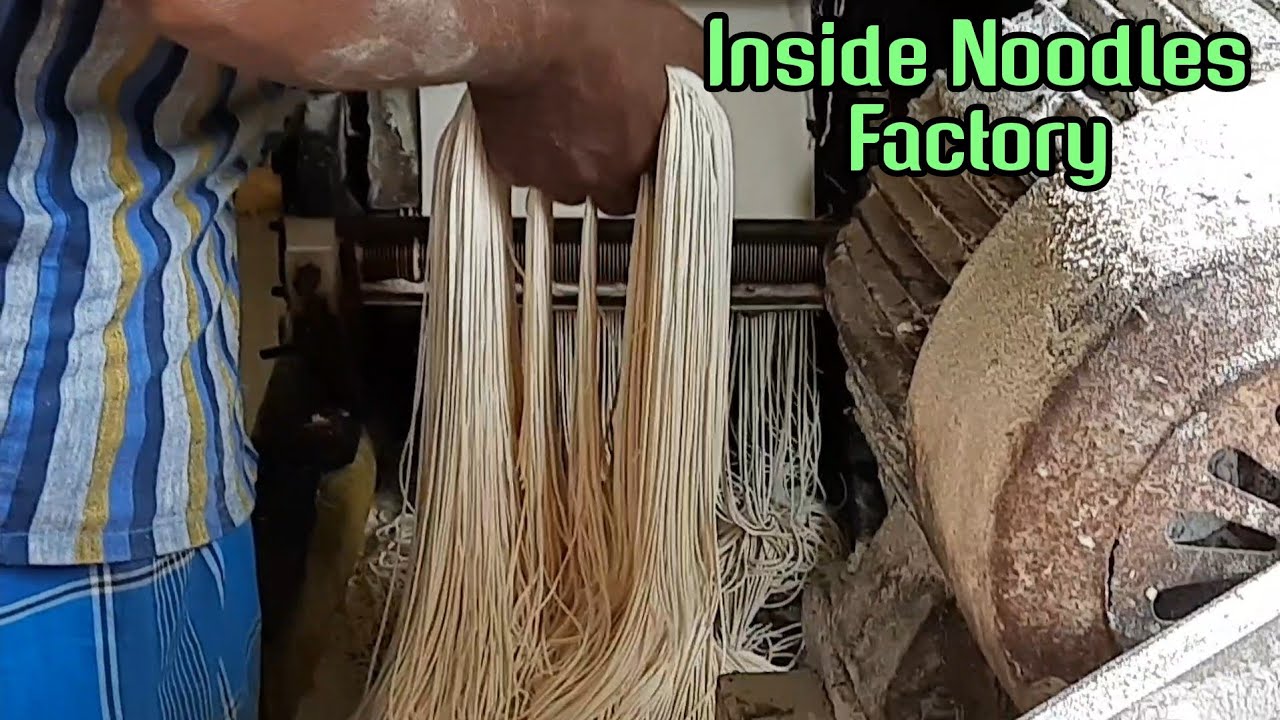The image depicts a close-up scene inside a noodle factory. In the top right corner, green text with a black drop shadow reads "Inside Noodles Factory." The focus is on a worker with light brown skin, partially covered in flour, seen from the side view on the left. Their arm extends from the top left, descending diagonally into the frame. They're wearing a shirt with vertical stripes in dark blue, light blue, yellow, and white, paired with plaid blue, white, and black bottoms. The worker's hand, dusted with flour, grasps a bunch of long noodles that hang downwards.

In the background, a machine processes the noodles. Flat dough enters one side and passes through a grooved, coiled cutting implement to emerge as thin strands of pasta. On the right side of the image is an old, possibly vintage, cylindrical piece of machinery with rusty, brownish sections and white stripes, covered in flour. The face of this machine has a grate with circular openings. The image captures a moment of manual noodle handling amid the mechanized process in an industrial setting.